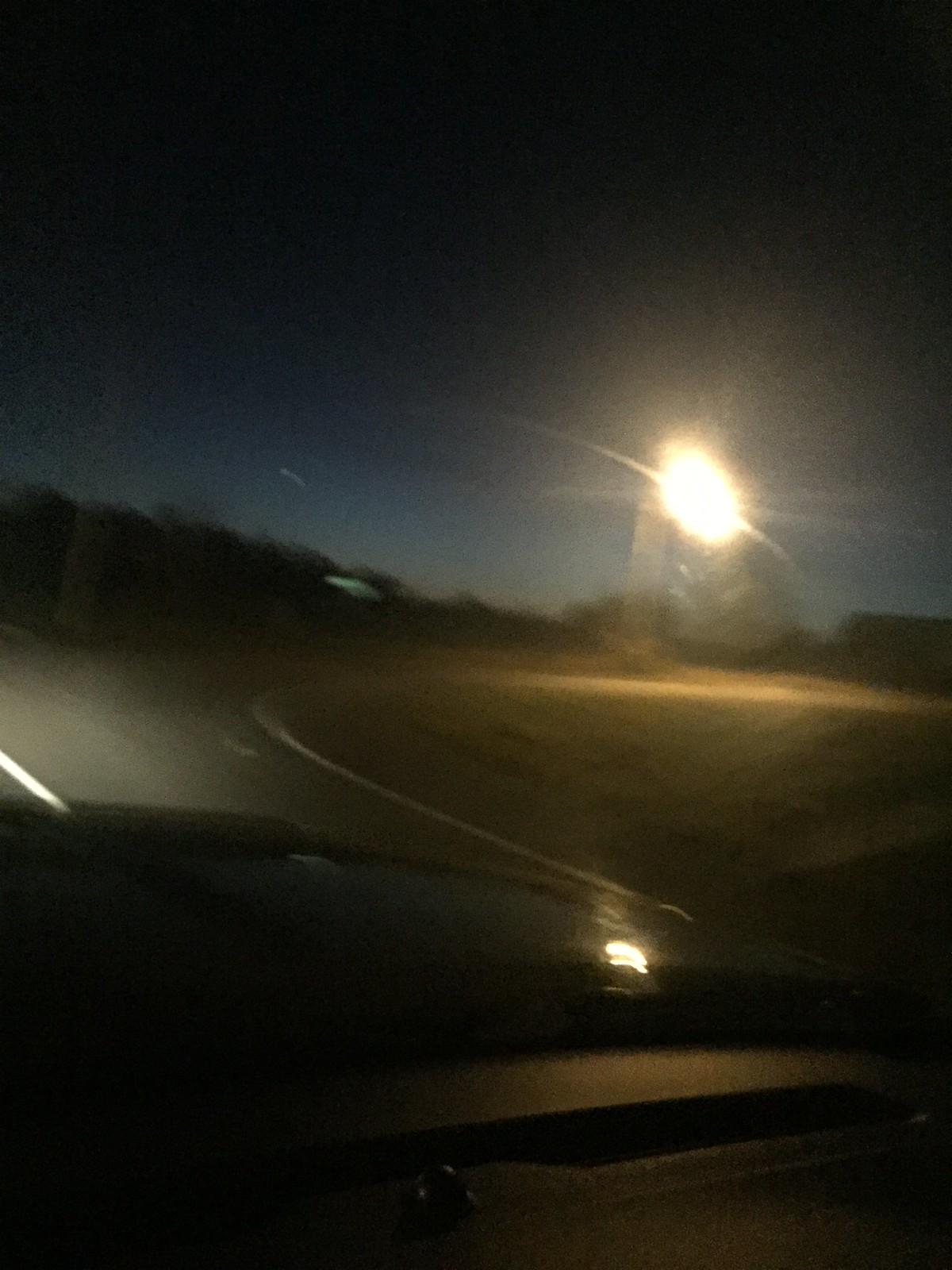Captured from the interior of a moving car, the photograph depicts a stark, luminous celestial body — potentially the moon or the sun during an eclipse — dominating the night sky. The intense brilliance casts a shadow across the front of the vehicle, while its reflection shimmers in the windshield. The car appears to be driving on a road that curves gently to the right towards a notable monument illuminated by the celestial light. Framed by a deepening twilight that nearly plunges into darkness, the scene includes silhouettes of nearby houses. Additionally, the car’s windshield wiper is faintly visible, adding a touch of realism to this mesmerizing, almost otherworldly capture.